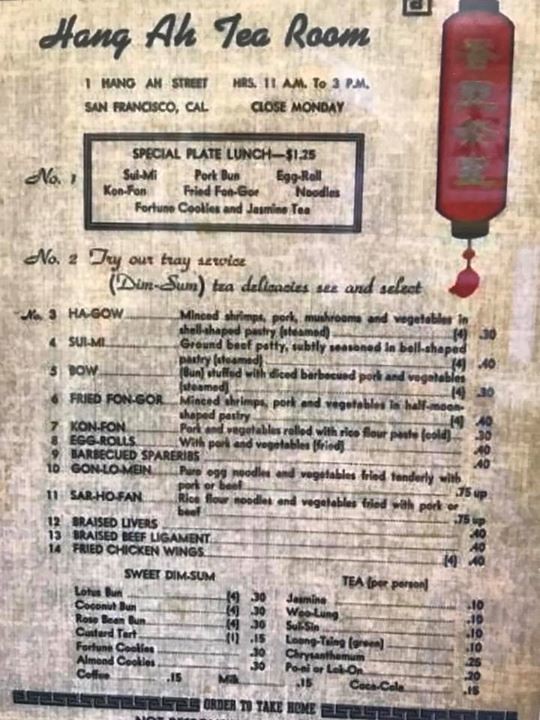Hang Ah Tea Room, located at 1 Hang Ah Street, San Francisco, California, showcases its operating hours prominently, noting that they are closed on Mondays. In the upper right-hand corner of the image, there is a traditional Chinese paper lantern adorned with Chinese characters.

At the top of the image, a black box highlights two special offerings. The first is the "No. 1 Special Plate Lunch" priced at $1.25, featuring a selection of dishes including sui mee, con fan, pork bun, fried fen gore, egg roll, noodles, fortune cookies, and jasmine tea.

The second offering invites patrons to try the tray service featuring dim sum and various tea delicacies. A detailed, a la carte menu of dim sum items follows, including:
- **Hao Gao**: Minced shrimp, pork, mushrooms, and vegetables in a shell-shaped pastry, steamed, 4 for 30 cents.
- **Sui Mee**: Ground beef patty subtly seasoned, in bell-shaped pastry, 40 cents.
- **Bao (Bow)**: Bun stuffed with sliced barbecue pork and vegetables, steamed, 30 cents.
- **Fried Fen Gore**: Minced shrimp, pork, and vegetables in a half-moon-shaped pastry.
- **Con Fan**: Pork and vegetables rolled in rice flour paste, served cold.
- **Egg Rolls**: With pork and vegetables, fried.
- **Gon Lo Mein**: Pure egg noodles and vegetables fried tenderly with pork or beef.
- **Sar Ho Fan**: Rice flour noodles and vegetables fried with pork or beef.
- Additional offerings include braised livers, braised beef ligament, and fried chicken wings.

Two columns at the bottom of the menu list sweet dim sum varieties and teas. The sweet dim sum includes:
- **Lotus Bun**
- **Coconut Bun**
- **Rose Bean Bun**
- **Custard Tart**
- **Fortune Cookies**
- **Almond Cookies**

Alongside, common beverages such as coffee (15 cents), milk (15 cents), and Coca-Cola (15 cents) are listed.

The tea selection, priced per person, includes:
- Jasmine
- Wo Long
- Siu Sin
- Long Cin
- Green
- Chrysanthemum
- Po Air
- Leek On

The entire menu is printed on a textured, light brown cream paper, providing a rustic and traditional feel to the presentation.